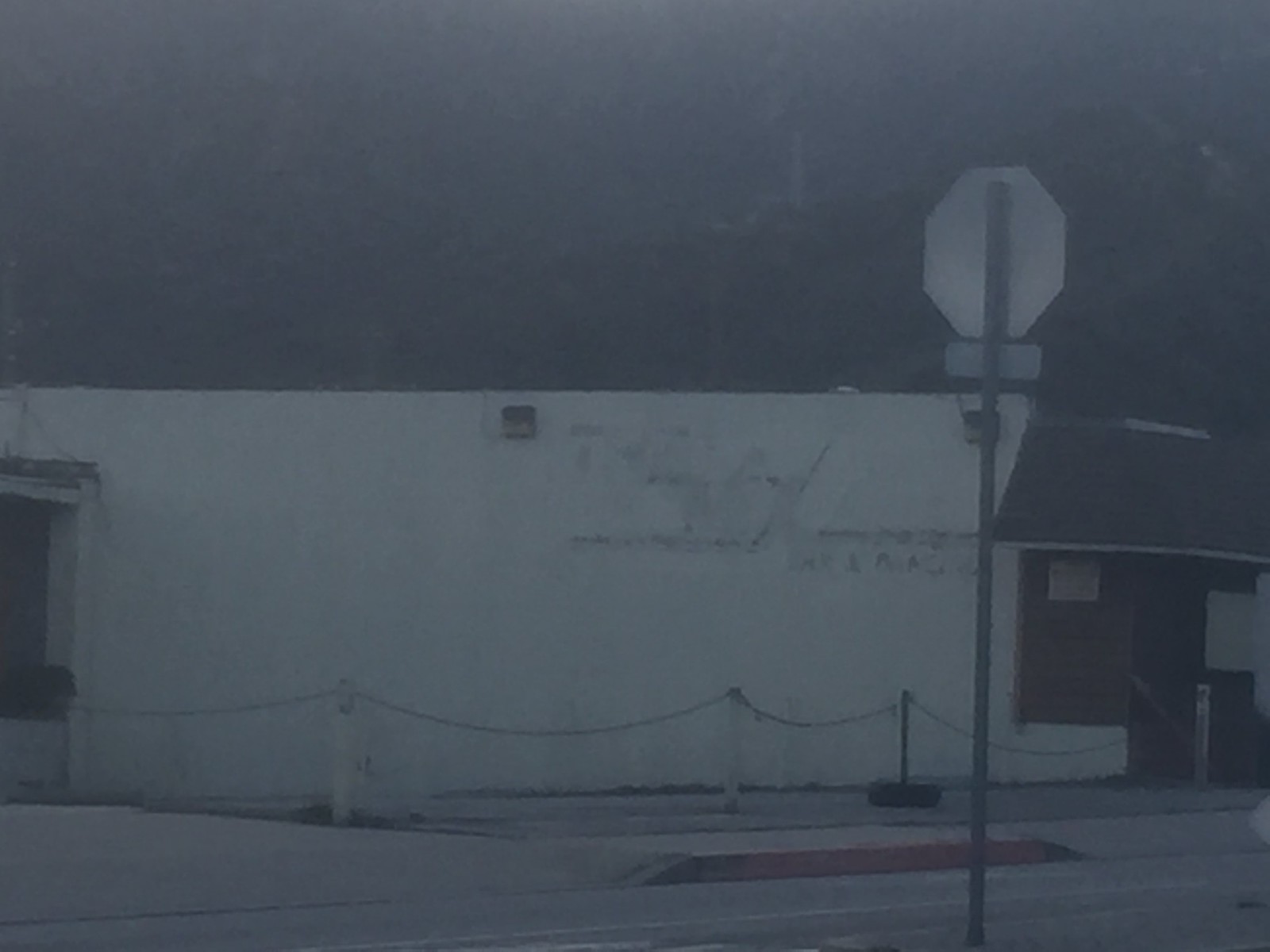A vacant store rests silently, indicating it may have gone out of business. The once-prominent store sign is now absent, leaving faint traces on the white wall that forms one side of the building. The parking lot is secured with a sturdy metal gate, extending from one support to another, hinting at a time when the lot buzzed with activity. Across the street, the back of a stop sign is faintly visible, adding to the somber scene. The entrance door is eerily boarded up, with no windows in sight, and a solitary sign tacked onto the wooden barricade. The image is captured in dim lighting, which casts an even more forlorn outlook on the surroundings. To the left, remnants of what appears to have been a loading dock add to the desolate atmosphere. In the background, towering mountains stand still, their presence underscoring the store's isolation.